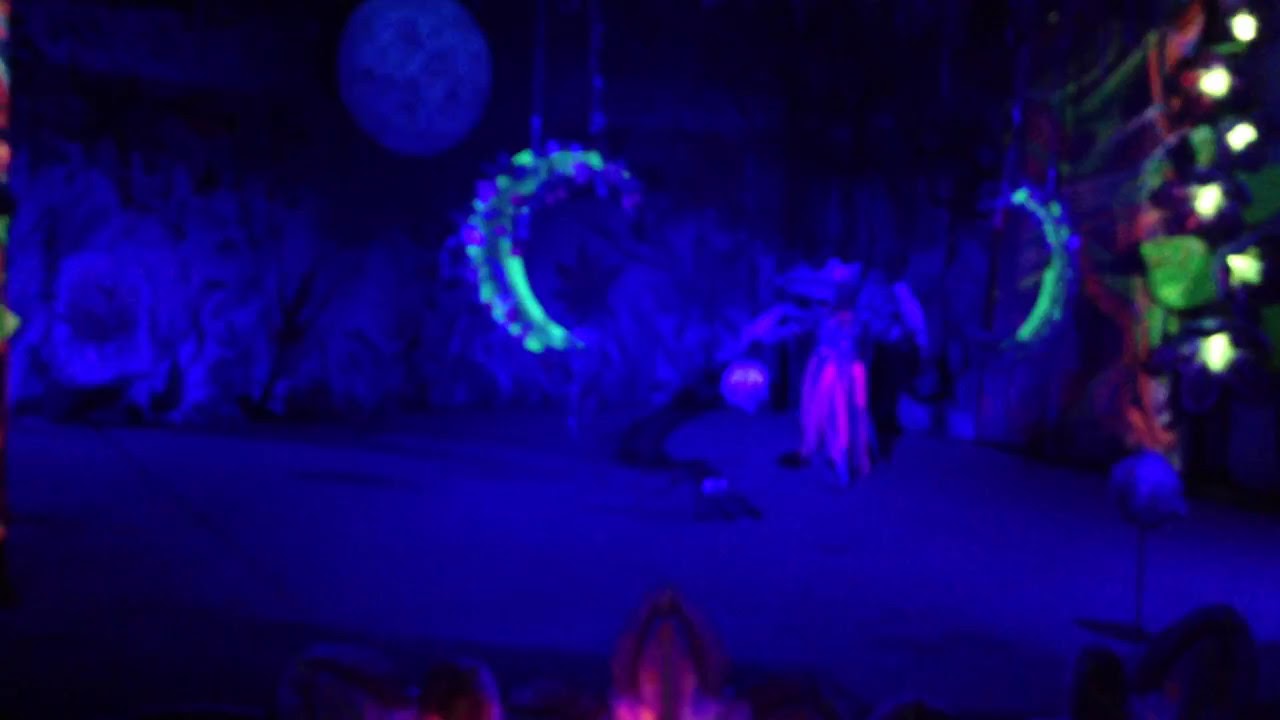This image is a blurred, color photograph taken from some distance, depicting a stage performance in a dimly lit auditorium. The landscape-oriented photo is dominated by dark and light blue hues, with the stage floor and background prominently featuring these colors. A couple of characters, possibly in costume, can be seen amidst the predominantly dark setting. One central figure seems to be dressed in a flowing white outfit with pink stripes, resembling a bird costume. The stage is enhanced by decorative elements, such as silver moons hanging on both sides and a prominent full moon illuminated in the upper left-hand corner. To the right, a strand of multicolored lights, which appear to be red, green, and blue along with white lights, stretches towards the ceiling, adding a vibrant touch to the scene. The lower forefront reveals hints of the audience, with partial views of their hands and heads. Despite the blurriness, the image conveys a rich, colorful atmosphere of a theatrical or ice performance.